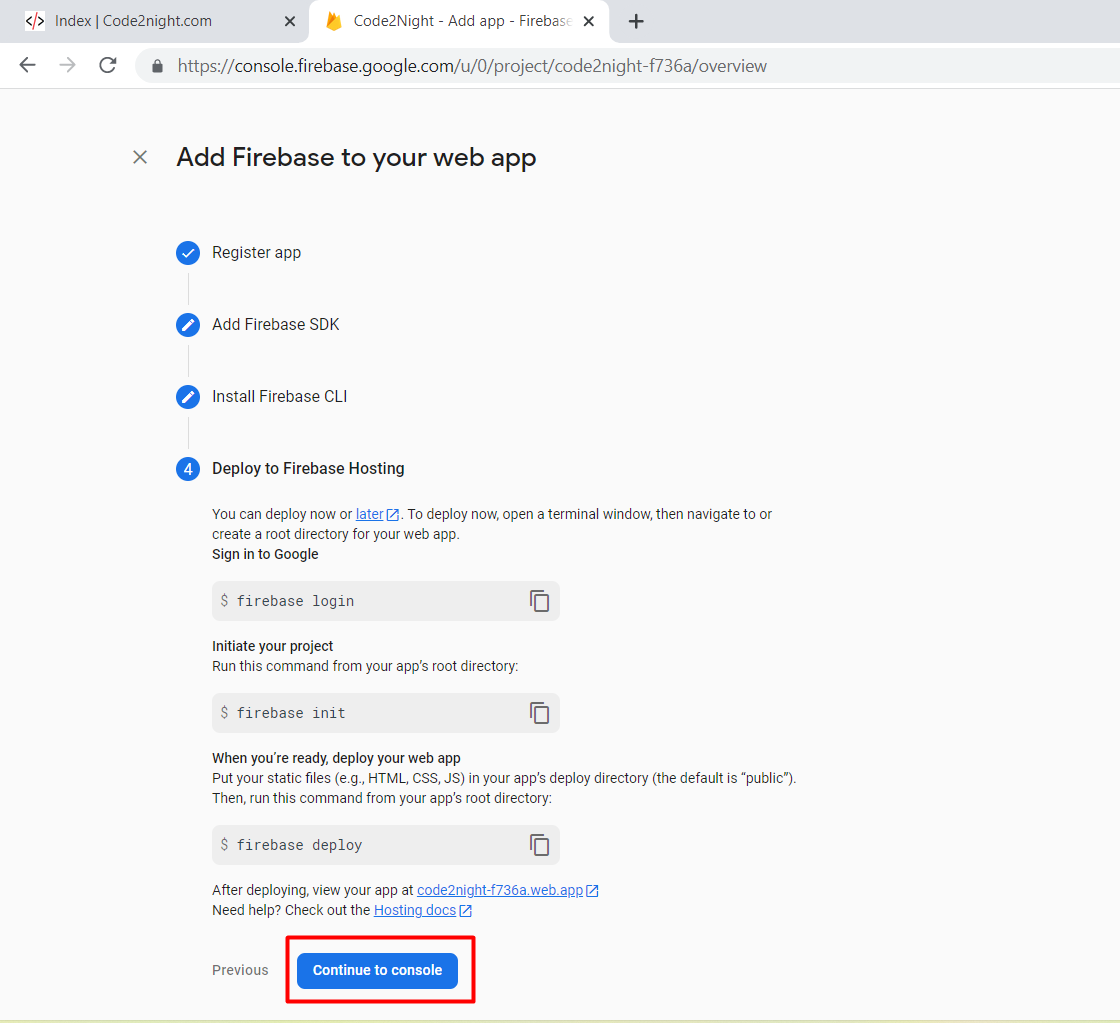The image portrays a section of a website interface, specifically a web application console from Firebase. At the top, a gray bar hosts two tabs. The first tab on the left is labeled "index code to night.com," while the currently active tab reads "Code to Night at app, console.firebase.google.com."

Beneath the tabs, a black header text reads, "Add Firebase to your web app," accompanied by a small 'X' icon for closing this section. The page is largely composed of a white or light gray background with black text, accented by blue icons and highlights.

The main content consists of a step-by-step guide in black text for integrating Firebase with a web application. The steps include:

1. **Register App:** A section with a blue checkmark indicating completion.
2. **Add Firebase SDK:** Accompanied by an editable option.
3. **Install Firebase CLI:** Also with an editable option.
4. **Deploy to Firebase Hosting:** Marked with a blue number "4." This section explains that deployment can be done immediately or later.

For immediate deployment:
- Open a terminal window.
- Navigate to or create a root directory for your web app.
- Sign in to Google using the command `Firebase login`.
- Initialize your project by running `Firebase init`.
- Prepare your static files (e.g., HTML, CSS, JS) in the deploy directory, defaulting to "public."
- Deploy the app using the command `Firebase deploy`.

Post-deployment:
- Your app will be accessible at a URL, denoted as "code tonight-f736a.web.app," which is clickable.
- For further assistance, a clickable "hosting docs" link is provided.

At the bottom of the page, a red rectangular button labeled "Continue to Console" urges the user to proceed, with a "previous" button next to it for navigation.

Overall, the layout is designed for ease of following the deployment steps, with clear instructions and clickable elements for further actions or help.